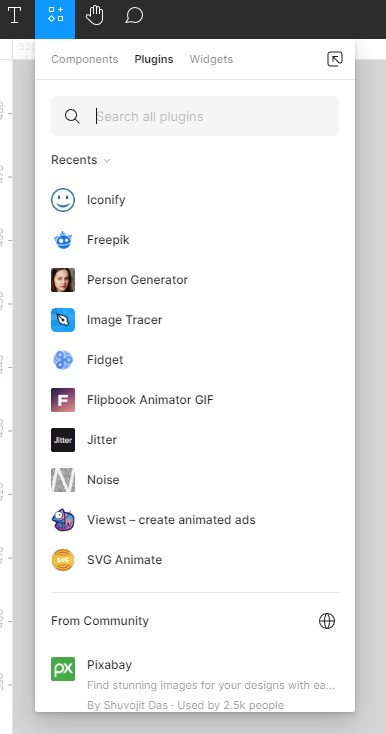The image is a detailed screenshot of a website interface. In the top left corner, there are four category icons: a white "T" icon, a set of four icons (two squares, a plus symbol, and a diamond symbol) highlighted in blue, a right-hand icon, and a chat bubble icon. Below these icons, there is a pop-up menu with three categories at the top: Components, Plugins, and Widgets, along with a share button icon to the right. Beneath these, there's a search bar labeled "Search all plugins" with a magnifying glass icon on the left. Underneath the search bar, the word "Recents" appears with a drop-down arrow next to it. A list of various app names follows in a vertical arrangement: Iconify, Freepik, Person Generator, Image Tracer, Fidget, Flipbook Animator GIF, Jitter, Noise, Views ST, and SVG Animate. This section is separated by a thin black line from another section labeled "From Community," which lists "Pixabay."